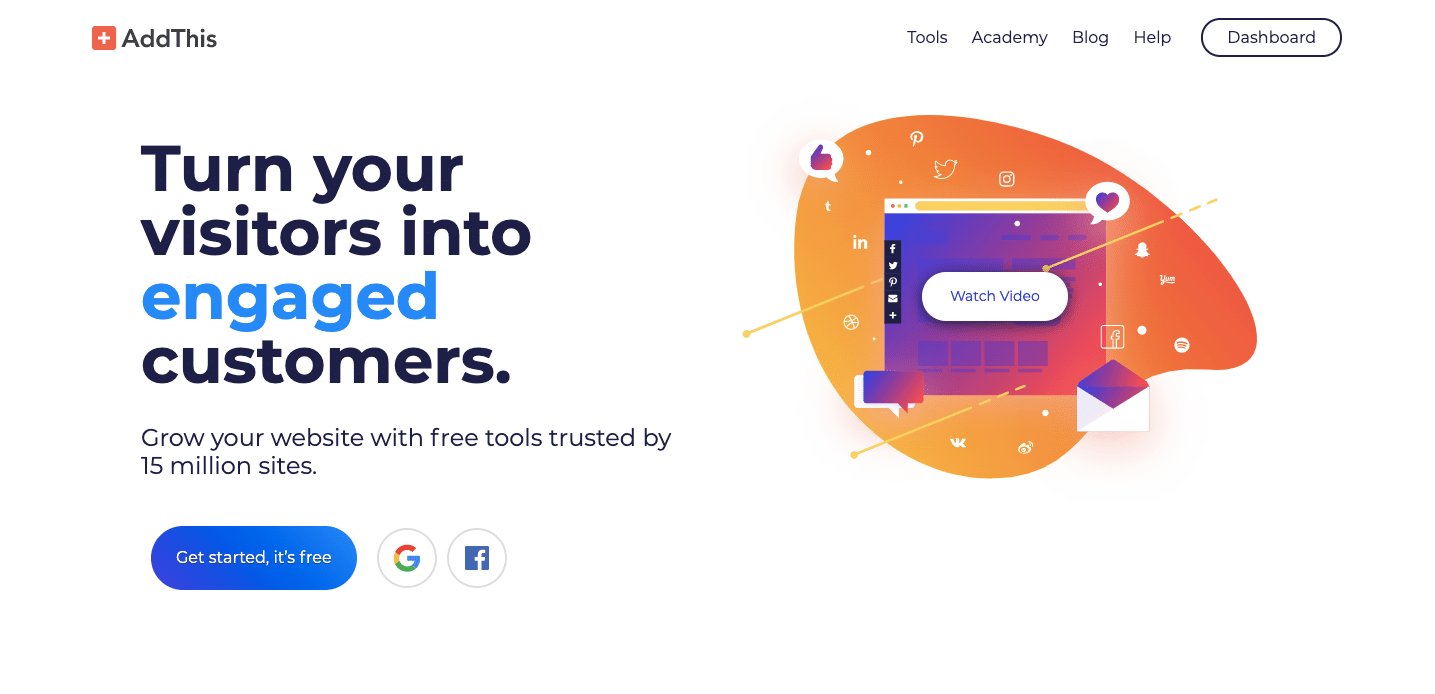The promotional image encourages visitors to add a specific website tool called "AddThis." The focal point is an orange square with a white plus sign at its center. On the left side, bold text reads, "Turn your visitors into," with the word "engage" highlighted in blue, followed by "customers." Beneath this, additional text states, "Grow your website with free tools trusted by 15 million sites."

A prominent blue button labeled "Get Started - It's Free" invites users to begin using the tool. Nearby, circular icons represent Google with its distinctive multi-colored "G" logo, and Facebook with a blue square and white "F" symbol.

At the top right corner of the image are navigation options: "Tools," "Academy," "Blog," "Help," and a circled "Dashboard." The dashboard icon resembles a paint palette, adding a creative touch.

Center stage is an option to watch a video explaining how the tool can enhance your website—depicted as a screen with "Watch Video" written in the center. The palette background is a vibrant orange, decorated with icons for various social media platforms like Pinterest, Instagram, and Twitter.

Additionally, the upper right corner features a heart split into pink and purple halves, while the upper left showcases a "thumbs up" symbol. A purple box with a gradient of purple and pink sits prominently in the center.